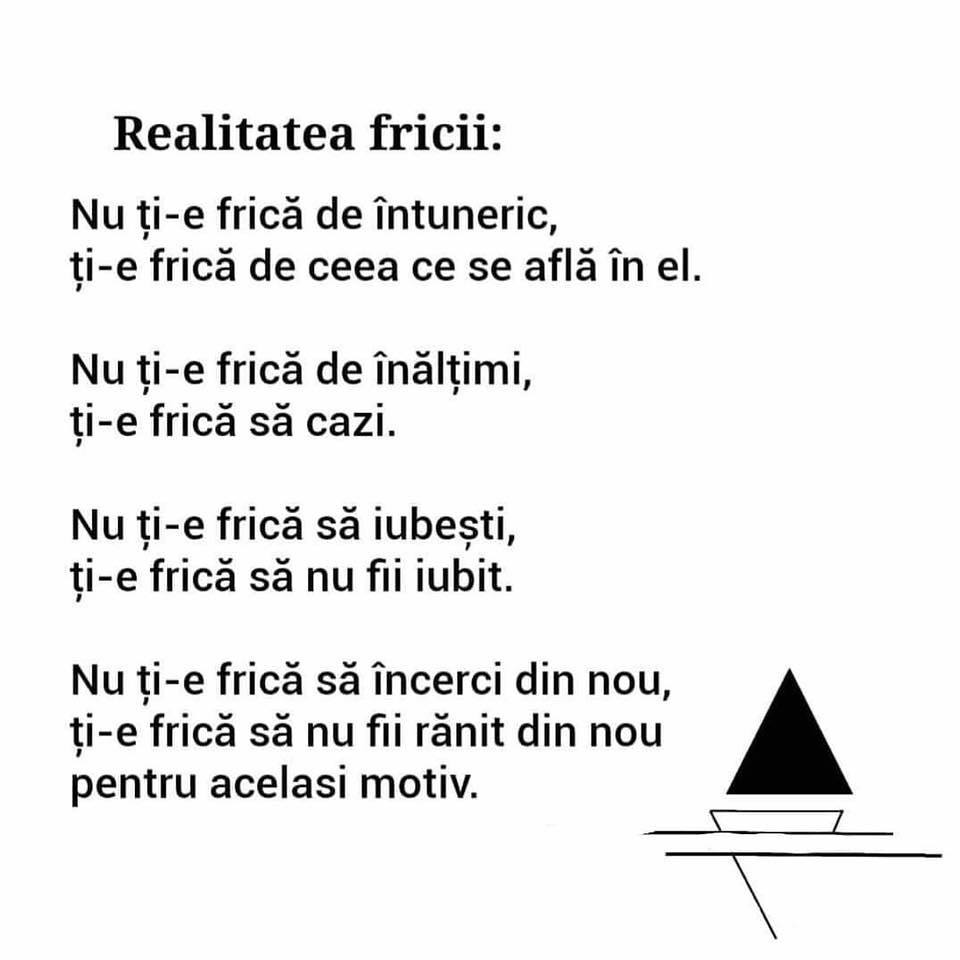The image displays a scanned page with multiple lines of text written in what appears to be Romanian, set against a white backdrop. The text is entirely in bold, black print. At the top, the title reads "Realitatea Fricii," followed by a colon. The various lines of text include numerous accented characters such as an A with an accent sign over it, an I with an accent sign over it, and a T with a sign beneath it. 

In the bottom right corner, a distinctive logo is present, consisting of a black triangle adjacent to a white triangle. The white triangle has one of its sides incomplete and features two lines intersecting in the middle, together forming a diamond-like shape with the bottoms touching.

The text content includes phrases broken down into individual words, punctuated with commas and periods for clarity. For example, one line reads, "Nu tie frica de intuneric," and another reads, "Tie frica de cee ce afli in el." These phrases explore themes reflective of the inherent fears associated with darkness and the unknown.